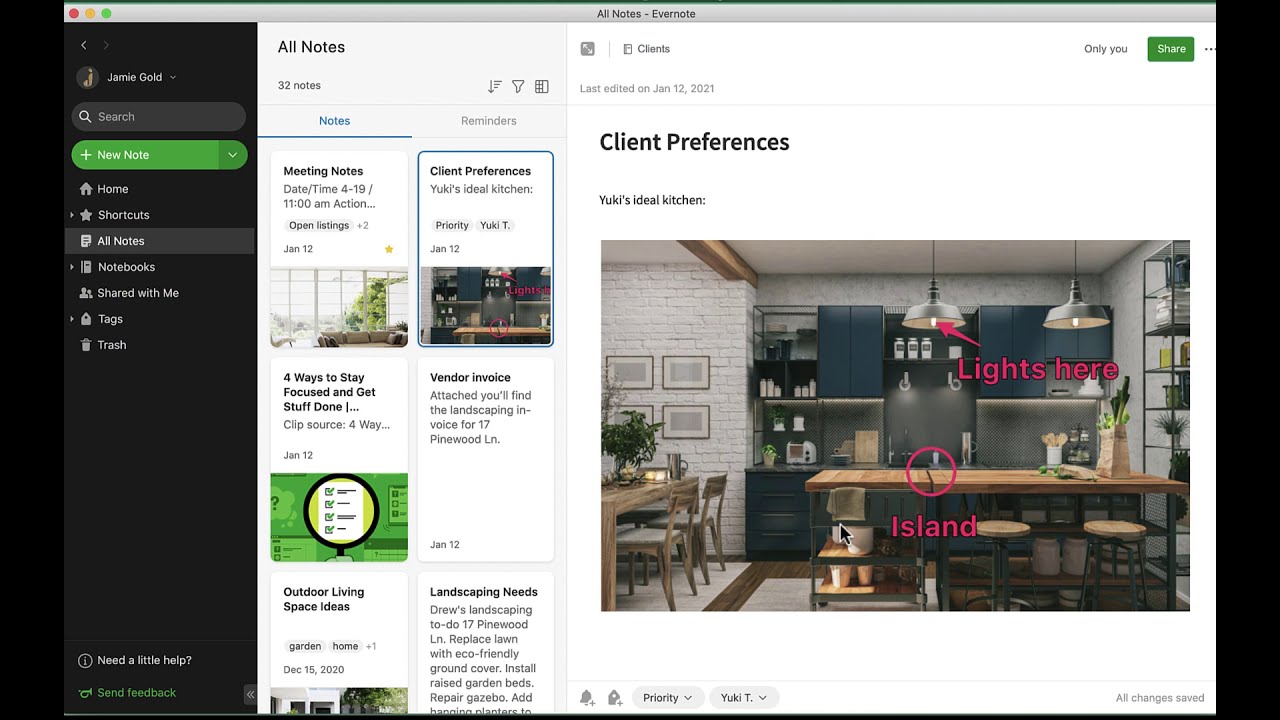This image is a screenshot from a computer displaying a page titled "Yuko's Ideal Kitchen," which was last edited on January 12th, 2021. The page contains sections for client preferences, new additions, and comprehensive notes. Prominently displayed is a photograph of a kitchen featuring a wooden island with a clearly marked seam where two tables have been joined, highlighted by a red circle. Overhead, there are hanging lights with black fixtures designed to direct light downwards, one of which is specifically pointed out by a red arrow. The interface of the page indicates various client-specific details and considerations for the kitchen setup.